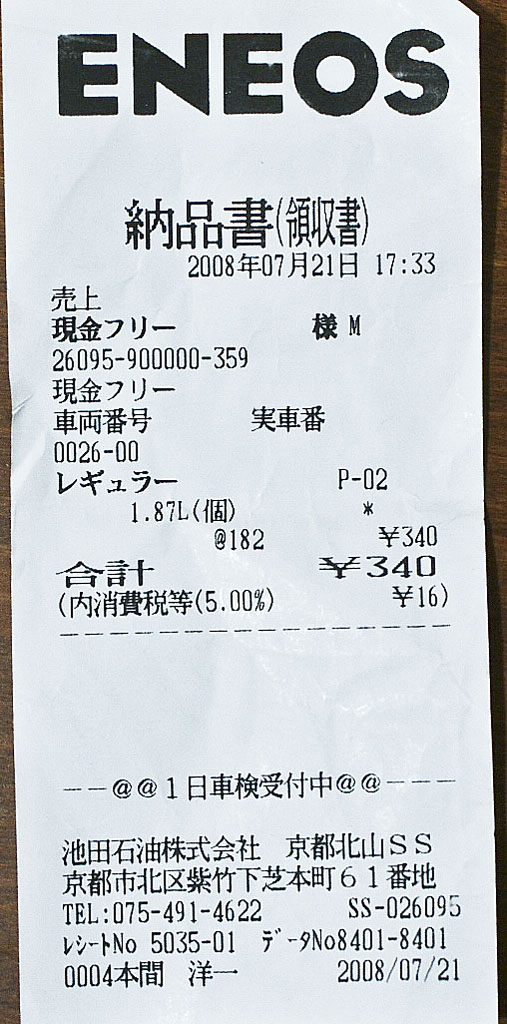A white receipt is prominently displayed against a stark black background. The text on the receipt is entirely in an Asian script, most likely Chinese or Japanese, printed in black ink. Despite the language barrier, a few details stand out: the date "2008-07-21" is clearly visible at both the top and bottom of the receipt, indicating that it is from July 21, 2008. At 17:33, presumably the time of the transaction, several items are listed. One notable entry indicates a purchase of "1.87 liters" costing "340 yen." Additionally, a tax of "5%" amounts to "16 yen." At the very bottom, the receipt bears a serial number or code: "SS-026095."